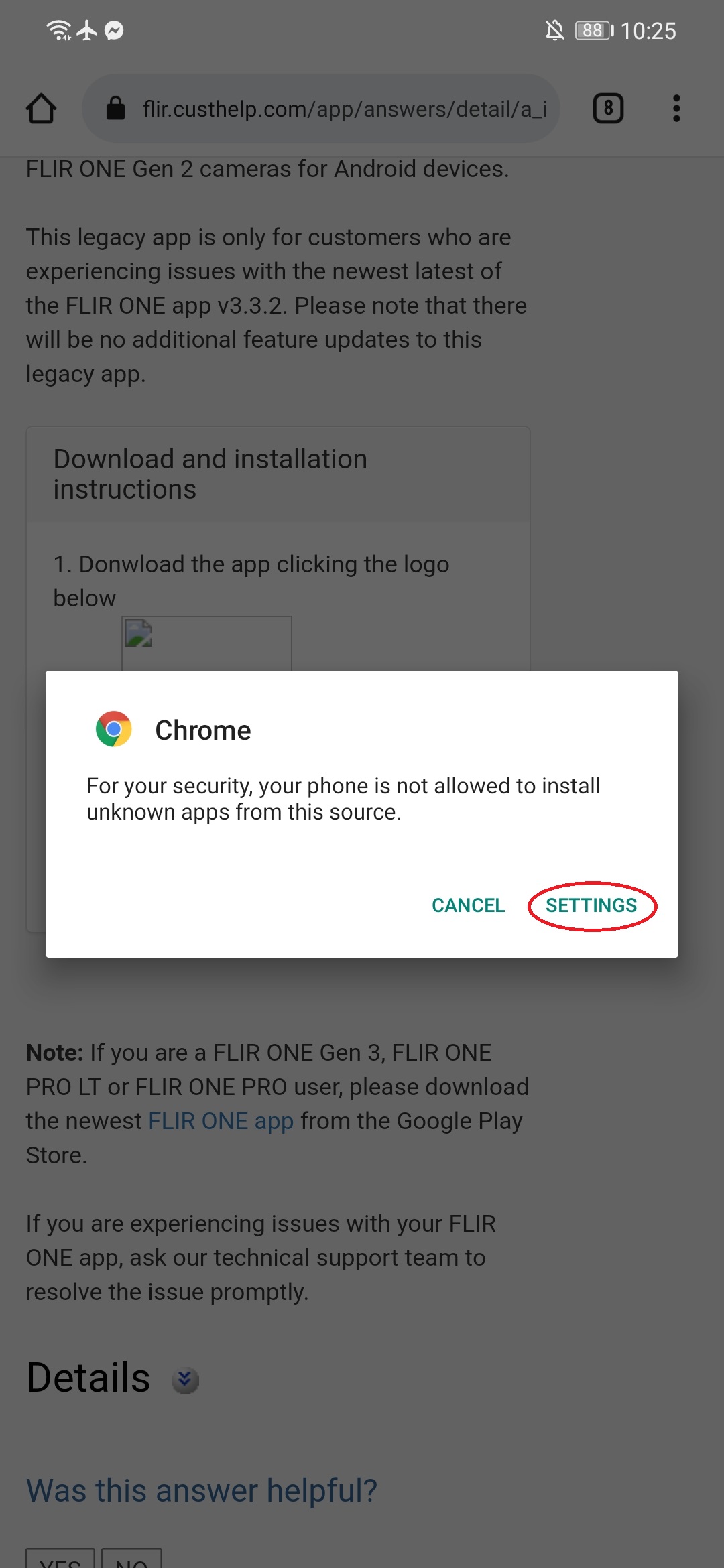The image displays a Google Chrome browser window with a prominent pop-up box indicating a security warning about an installation attempt. The pop-up box states, "Your security settings do not allow this application to be installed on your device," and offers a solution by directing the user to their settings, which is highlighted with a red circle. The background of this pop-up is greyed out.

In the browser window behind the pop-up, the website (flaired.co.za) appears partially visible. The page details information about the FLIR ONE Generation 2 cameras for Android devices, specifically noting that the legacy app is available for customers experiencing issues with the latest version. The website emphasizes that no additional features will be added to the legacy app.

Displayed prominently on the webpage are steps advising users to download the app, with a specific mention for users of FLIR ONE Gen 3, FLIR ONE LT, or FLIR ONE Pro to download a different app via a given blue hyperlink. Below this information, there is a section titled "Details" in bold black text, followed by a feedback prompt in blue text asking, "Was this answer helpful?" with options for users to select "Yes" or "No" to provide feedback for website improvement.

Additional details in the browser interface include an open tabs indicator at the top of the window, the battery life at 88%, and the current time displayed as 10:25.